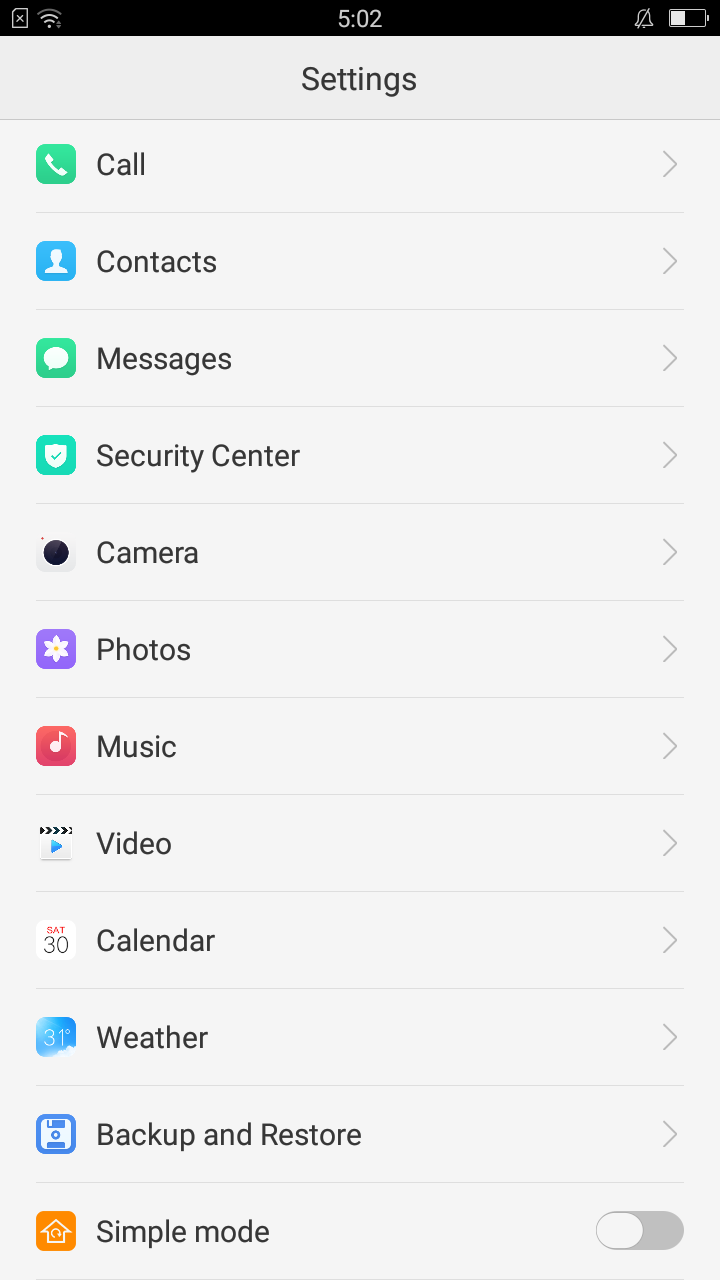A detailed mobile screen capture displays a settings menu, likely from a phone or an app. The top taskbar indicates the screenshot was taken at 5:02, displaying various status icons and showing the battery at slightly below 50%. The background is gray with the word "Settings" prominently centered in dark gray text. Each settings option is set in rows divided by thin, slightly darker gray lines. Each row features a minimalist icon on the left with a corresponding text label, and a small arrow button on the far right to navigate to detailed settings.

The list of categories from top to bottom includes: 
- Call
- Contacts
- Messages
- Security Center
- Camera
- Photos
- Music
- Video
- Calendar
- Weather
- Backup and Restore
- Simple Mode (with a toggle currently set to off).

The icons are minimalist, featuring solid color backgrounds with white symbols. They range in color from greens and blues to purples, reds, and oranges, giving a clean yet vibrant look to the interface.